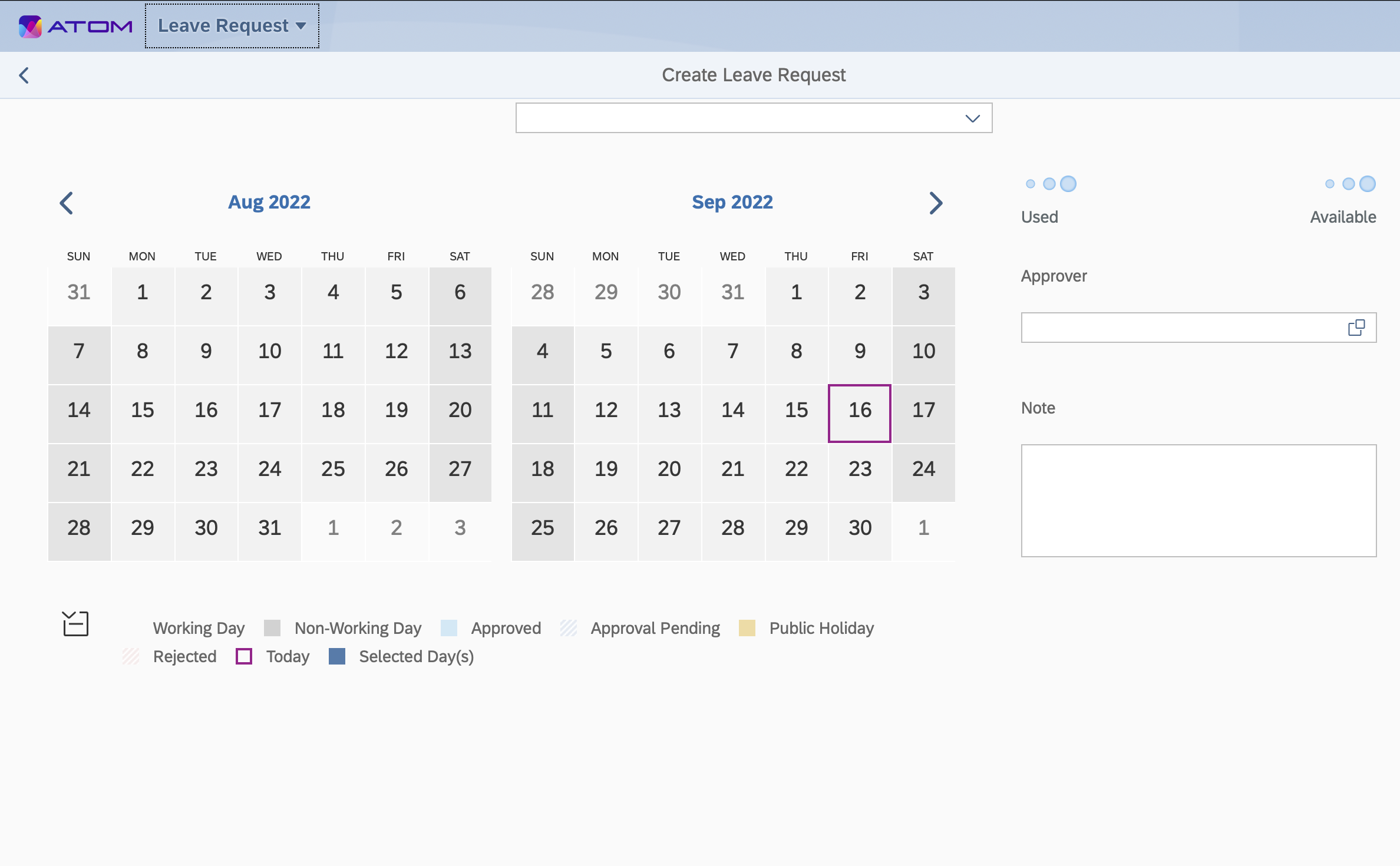This screenshot depicts a user interface from an application with an intricate and detailed layout primarily focused on leave requests and calendar functionalities.

In the top left corner, there is a multicolored square divided into five horizontal bands: dark purple, dark blue, pink, hot pink, and orange. This colorful square sits on a dark blue rectangle background. Directly to the right in purple text, it says "Adam a to M."

Below this, a rectangle with a black border encloses text written in dark blue that reads "Leave Requests" accompanied by a drop-down arrow. Adjacent to this, there's a lighter blue section with a left-pointing dark blue arrow, and centered text in white that states "Create Leave Request." Inside this section, a light gray rectangle contains a white drop-down arrow in blue.

Further down, two calendar views are displayed. The first calendar shows August 2022 with dates ranging from 31st of July to the 3rd of September. The days of the week are listed in all caps: "SUN," "MON," "TUE," "WED," "THU," "FRI," and "SAT," with a blue arrow indicating navigational control to go back. Specific dates are marked with varying shades of gray: 
- Dark gray bands encompass 7, 14, 21, and 28 of August, 
- Another dark gray band includes 6, 13, 20, and 27 of August, 
- Mid-gray covers 1-5, 8-12, 15-19, 22-26, and 29-31 of August.
- Off-white gray mix highlights 1-3, and 31 of August.

The adjacent calendar for September 2022 maintains a similar setup. The month is denoted in bold, dark blue, hyperlinked text. Dates under "SUN" and "SAT" are notably marked:
- Dark gray underlines include Sundays: 4, 11, 18, 25 and Saturdays: 3, 10, 17, 24.
- Mid-Grays phase 1-2, 5-9, 12-16, 19-23, and 26-30.
- The 16th is selected with a distinctive purple border, while several dates like the 28-31 of August appear in an off-white gray.

A legend underneath explains various square color codings:
- A working day marked in black-text.
- Non-working day denoted by a gray square.
- Approved leave indicated by a light blue square.
- Approval pending shown with a white square, blue stripes.
- Public holiday displayed through a cream-colored square.
- Rejected leave symbolized by a purple square, associated also with "Today."
- Selected days represented by a dark blue square with "S/A" in parentheses.

To the far right, icons featuring three ellipses transition from small to large in dark blue with "used" labeled beneath in black for usage metrics. Similarly, another set of ellipses with "available" below depicts available metrics.

Just slightly further down, there is a section labeled "APPROVER" in full black text, alongside a white rectangle containing a dark blue square and another floating above it. Below this, the word "Note" appears in full black text above a large white rectangular input area.

This detailed user interface allows for comprehensive leave management and navigational clarity with a robust and color-coded visual guide.